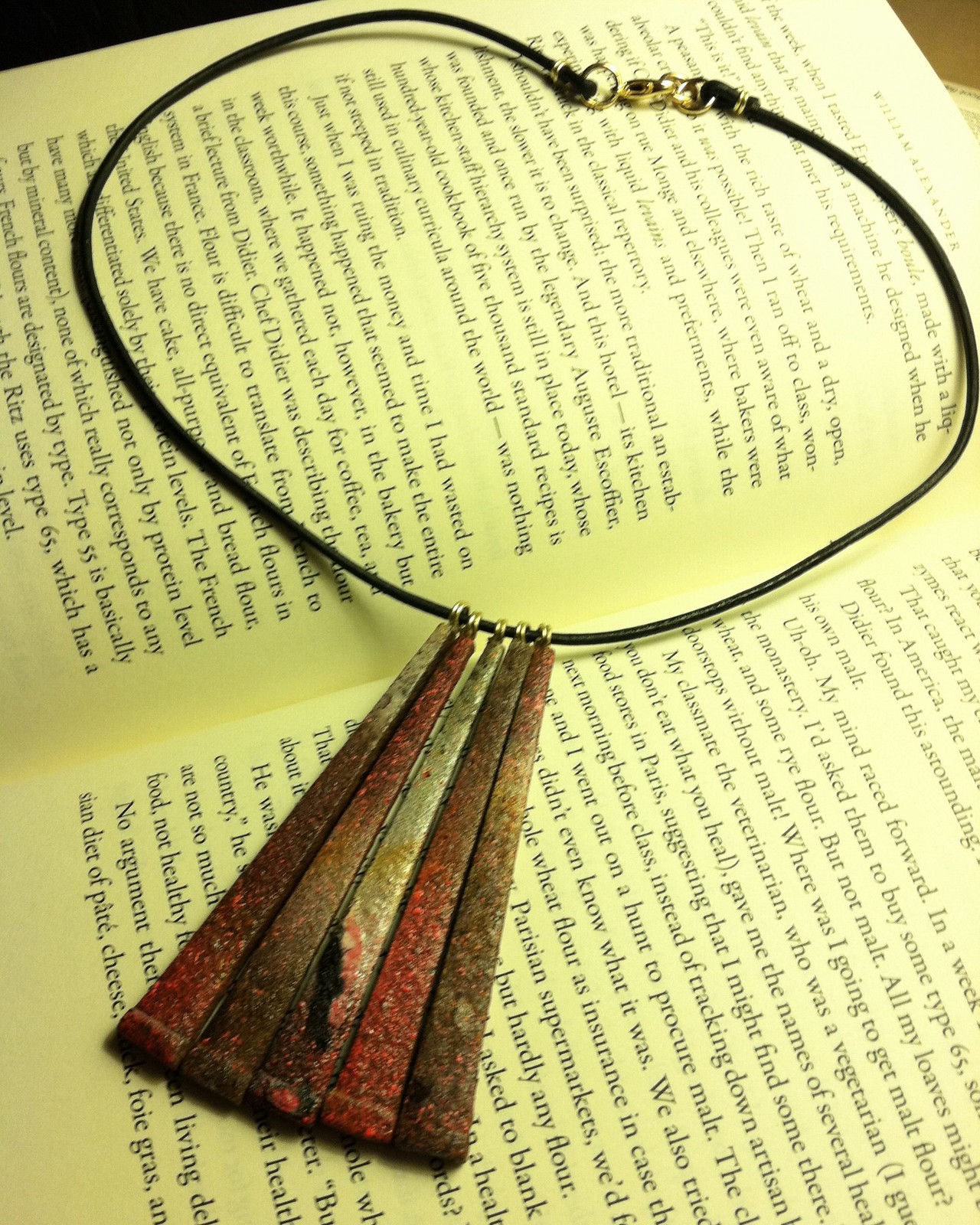This image features a vertically angled open book, with its off-white pages filled with dense black text. At the top of one page, the name "William Alexander" is prominently displayed, suggesting the author of the book. Placed atop the open book is a distinctive necklace with a thin black band and a silver clasp located at the upper center of the frame. The necklace, resembling a homemade piece, features five elongated triangular pendants hanging from it. These pendant shapes vary slightly in color, displaying shades of rust, reddish-brown, and browns, potentially crafted from stone or metal. Each pendant is attached to the necklace with small silver rings and widens gradually towards the ends, giving them a feather-like appearance. The unique combination of the rustic necklace and the vintage-looking book creates an intriguing and somewhat peculiar visual contrast.